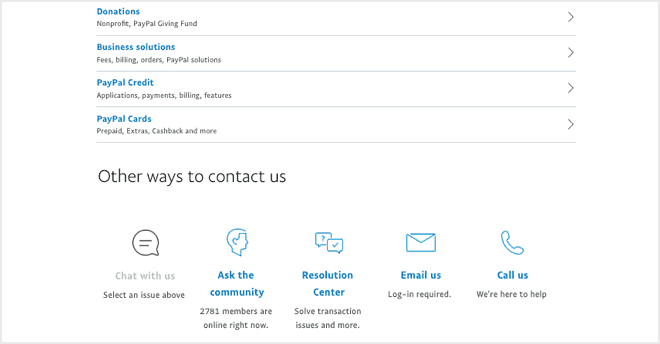The image features a white background bordered by a grey frame on all sides. At the top, bold blue text reads "Donation," followed by black text reading "Non-Profit PayPal Giving Fund." Below this, a dividing line separates the sections. The next line, again in blue text, states "Business Solution," followed by black text that reads "Fee Billing Order PayPal Solution." Another line appears beneath this.

Further down, in blue text, it says "PayPal Credit," followed by black text listing "Application Payment Billing Feature." A similar dividing line is placed below. Next, in blue text, "PayPal Cards" is written, with black text underneath listing features like "Prepaid Extras Cashback and More." Another dividing line follows.

Towards the bottom, a black text section in larger font declares, "Other Ways to Contact Us." Here, there are multiple icons and options for support. A chat bubble is labeled "Chat with Us" and directs users to select an issue from above. A profile silhouette icon labeled "Ask the Community" indicates that 2,781 members are currently online.

A text box with a question mark and another with a check mark are labeled "Resolution Center Solve Transaction Issues and More." Lastly, an envelope icon, requiring a login, offers the option "Email Us," while a phone icon reads "Call Us, We're Here to Help."